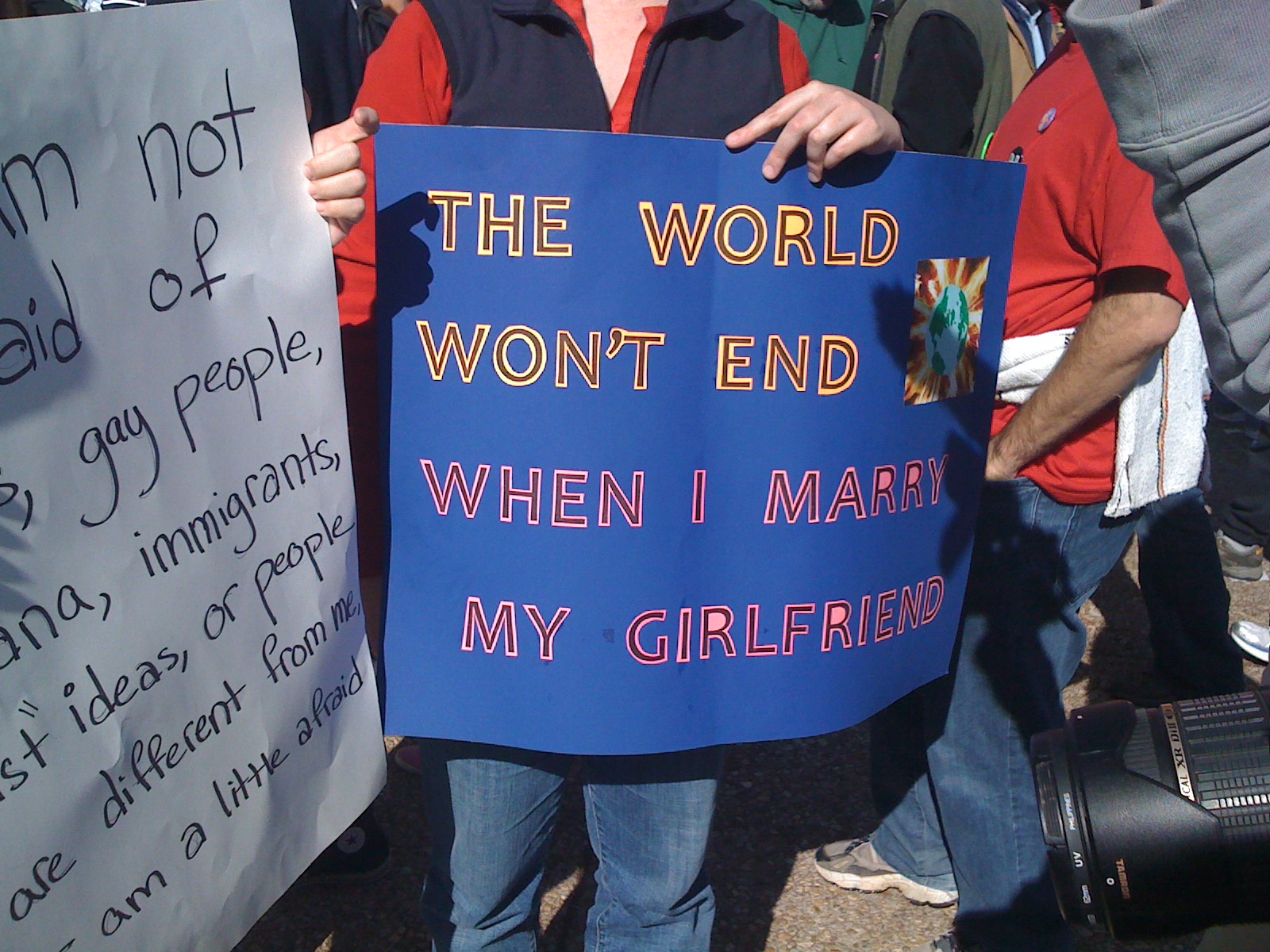The photograph is a close-up of a protest scene, capturing the torso and legs of participants, with a focus on two prominent signs. At the center, a person dressed in a red and black jacket holds a blue cardboard sign featuring bold black and yellow text that reads, "The world won't end when I marry my girlfriend." To their left, another larger homemade sign, white with handwritten black text, partially addresses issues involving immigrants and LGBTQ individuals, although not all the text is fully visible. The crowded environment showcases various figures, including a person in a red shirt with a sweater wrapped around their waist, looking off into the distance. In the bottom right corner of the image, a camera lens and a gray sweater sleeve are partially visible, alongside the feet of the protestors.